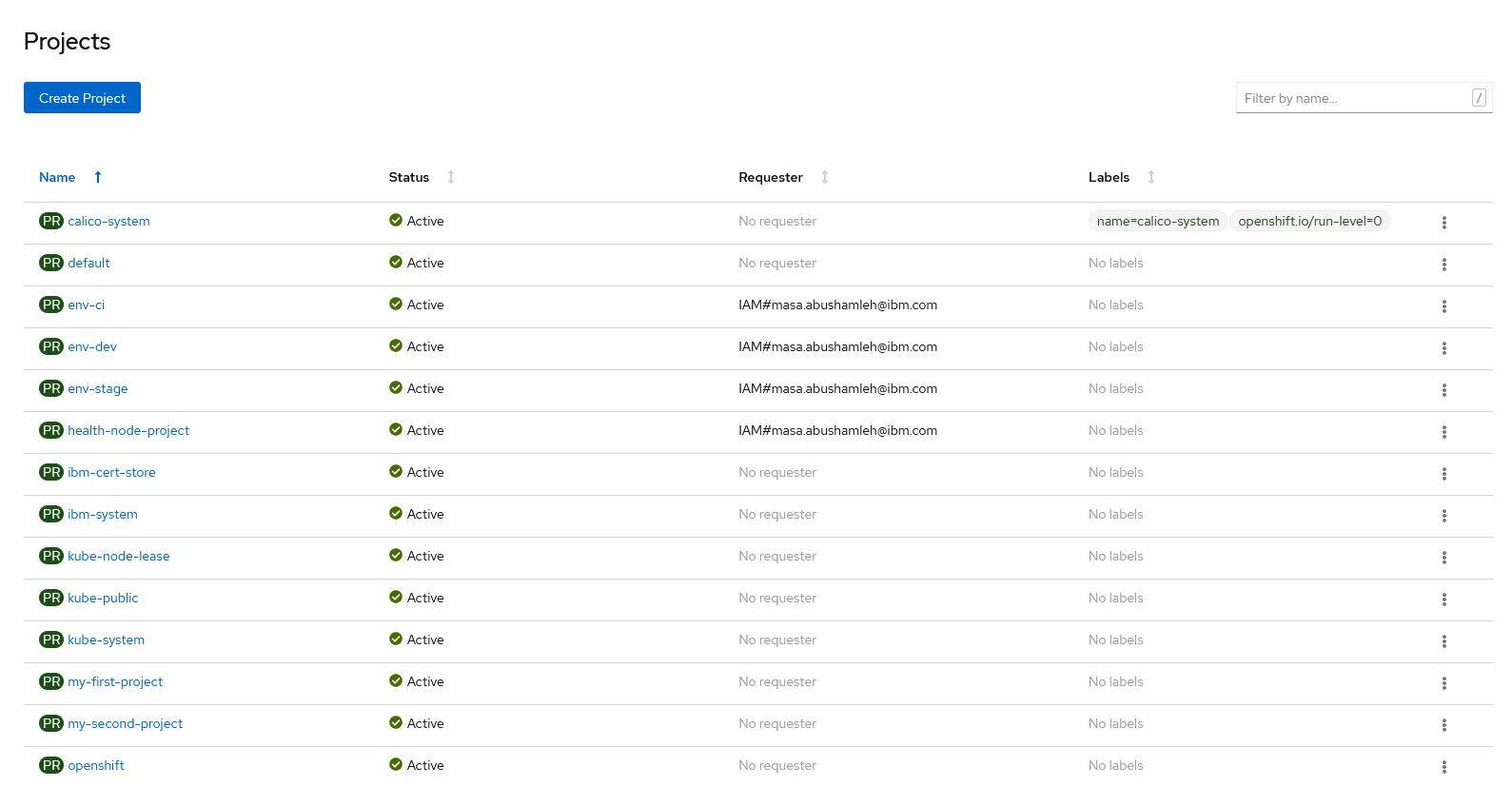**Detailed Caption:**

The screenshot displays a project management interface set against a white background. At the top, there is a blue rectangle with the label "Create Project." Next to it, a search bar is provided with the placeholder text "Filter by name."

Below the search bar, the interface is organized into columns with headers: "Name" (highlighted in blue with an upward arrow indicating ascending order), "Status" (displaying the statuses through green circles with white arrows), "Requester," and "Labels."

The first item listed is "Cisco System," shown in blue under the "Name" column. It has no requester listed and two labels associated with it. Following this, several project lines are displayed, but they all lack additional labels under the "Labels" column. 

One project entry reads "CNV" under the "Name" column, accompanied by an email address listed under the "Requester" column.